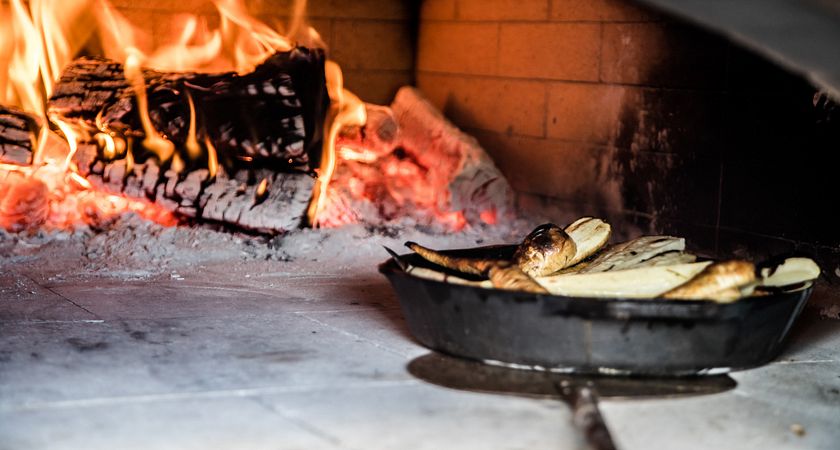This photograph, set in a horizontal rectangular frame, captures a rustic camping scene focused on the theme of cooking over an open fire. In the right foreground, a cast iron skillet brims with cooked food, possibly fish, displaying light cream and off-white hues with blackened, charred edges that slightly overflow the pan. Behind this, a vibrant wood fire burns within a red stone wall, casting warm light onto the setting. The fire extends beyond the confines of a makeshift fireplace composed of charred black logs with white ashy patches. The active flames rise high, mingling with glowing orangish coals nestled between the logs. To the left, a fire pit appears to be in use, contributing further to the overall atmosphere of heat and rugged outdoor cooking. The scene is set atop a white tiled floor, enhancing the contrast and detail of the elements within this compelling image.